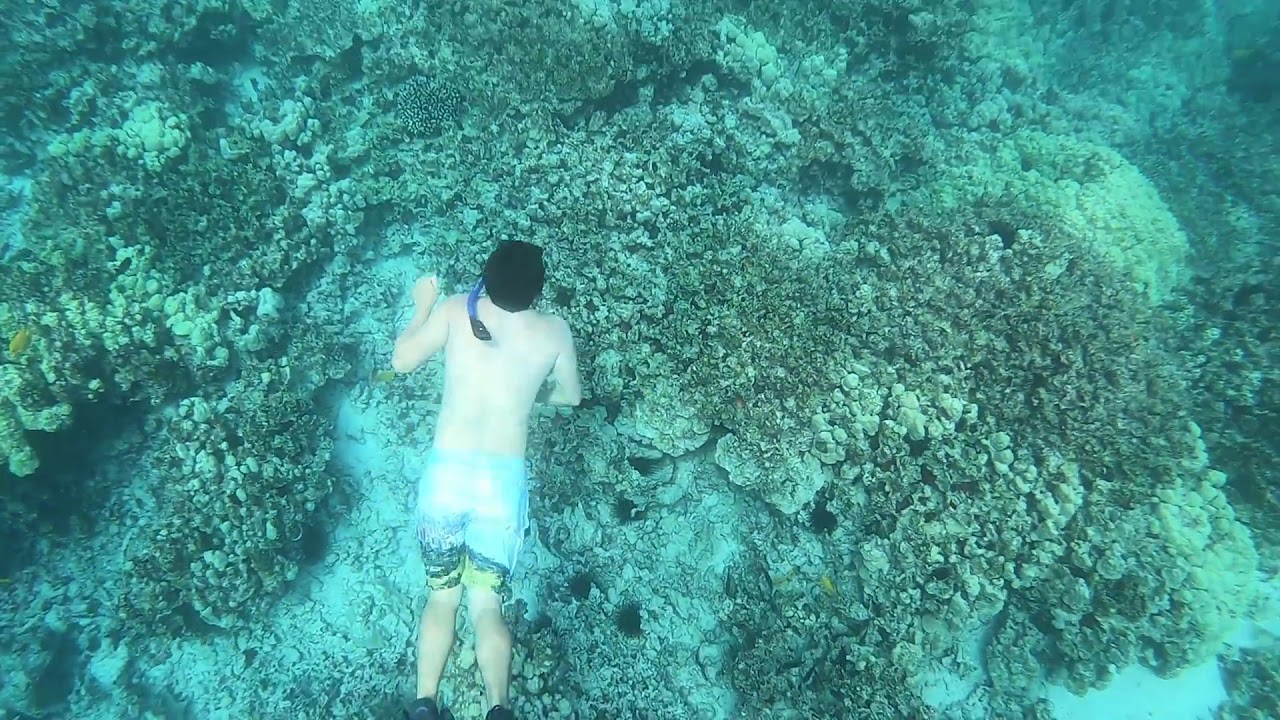This image presents an underwater scene viewed from above, showcasing a male snorkeler in an expansive oceanic space. The scene is dominated by various hues of green and aqua, giving a sense of depth and a watery atmosphere. The snorkeler, positioned in the left third of the image, is shown bare-chested, with dark hair, and wears blue swim trunks featuring a sky-like pattern. He has a snorkel, colored blue with a black tip, extending over his left side. His black flippers are just visible behind him. The ocean floor beneath him is lined with a large coral reef, characterized by its rough, gray, rock-like appearance and interspersed with mossy seaweed and other plant life. The overall palette includes shades of green, white, and light blue, emitted an aquatic overtone. Notably, the scene is free of any fish or underwater vehicles, focusing instead on the tranquil complexity of the submerged environment and the solitary figure exploring it.